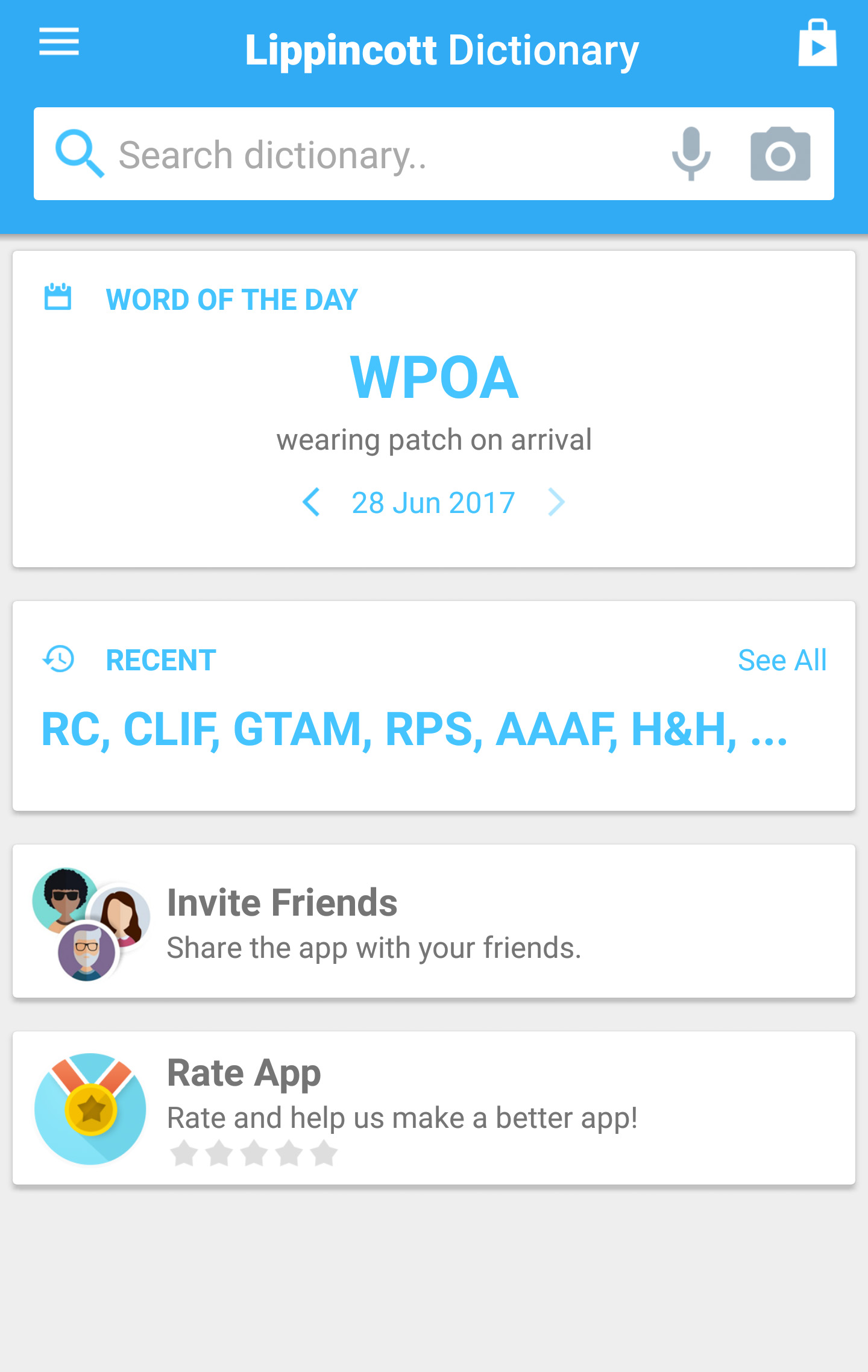The image displays a dictionary application screen titled "LIPNICOT Dictionary," with the name incorrectly spelled as L-I-P-P-I-N-O-C-O-T-T. At the top of the screen, there is a blue navigation bar containing a white search bar, featuring an icon with three lines on the left, likely a settings menu, and a bag with a play button on the right. The search bar itself includes microphone and picture icons.

Below the navigation bar, there's a "Word of the Day" section displaying the word "WPOA," which stands for "Wearing Patch on Arrival," followed by the date, June 28, 2017. Under this, there is a "Recent" section listing abbreviations such as RC, CLIF, GTAM, RPS, AAAF, and H&H, with a button offering to "See All" recent entries.

Further down is an "Invite Friends" section encouraging users to share the app, followed by a "Rate App" section prompting users to rate the app with a set of five gray stars. The app's design features a clean color scheme primarily consisting of white and gray, with blue accents, especially in the search bar area. The platform for the application is not specified, so it may be available on both iOS and Android.